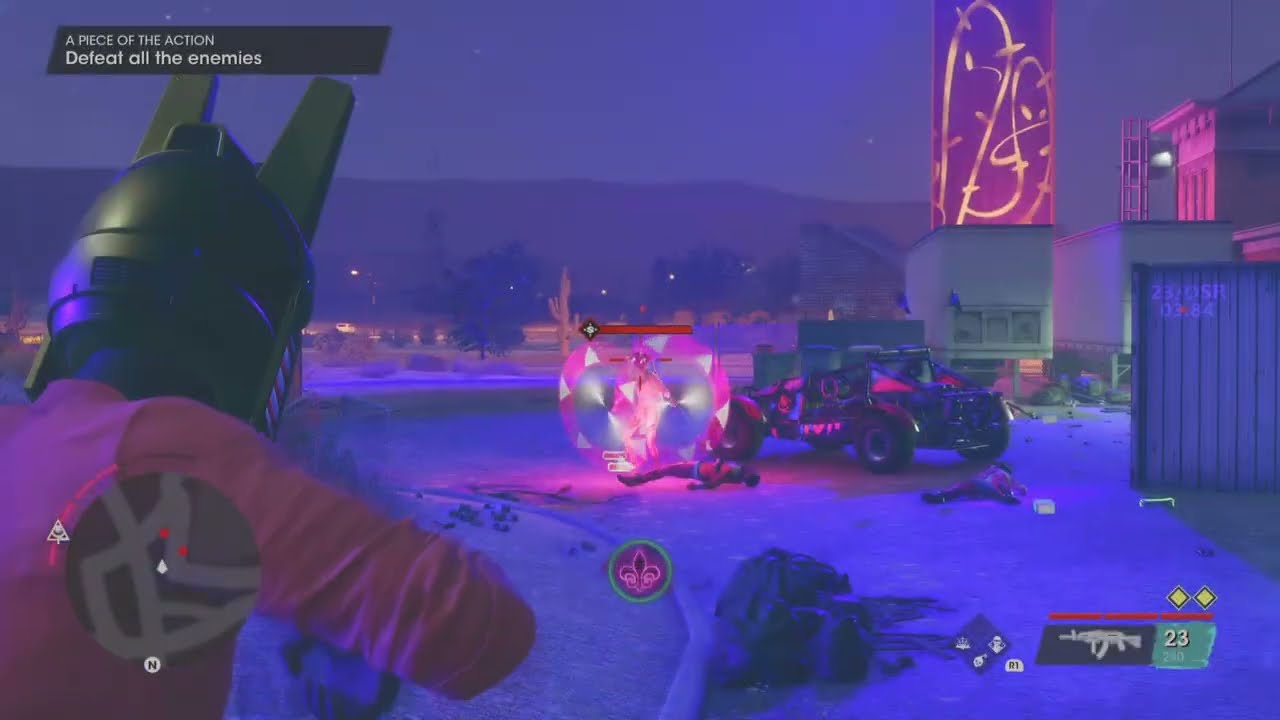The image is a detailed, rectangular screenshot from a video game with a cartoonish style and unnaturally bright colors dominated by blue and purple hues. Set in an industrial, snowy nighttime environment, the scene features an array of shipping crates, semi-trailers, and a central jeep-type vehicle. In the lower left-hand corner, the back of the main character is seen in third-person view. They are wearing a pinkish-purple top and a distinctive black helmet with spikes and ridges. They appear to be aiming a weapon at an enemy standing near the jeep. The enemy character, bathed in pink and adorned with an aurora-like pink and white helmet, is positioned centrally in the image. Above, an apparent caption reads "A piece of the action. Defeat all the enemies," while a purple vertical rectangle with elegant gold wavy lines decorates the top right corner. In the background, snowy mountains loom beneath a nighttime sky, contributing to the game's vibrant and immersive atmosphere.